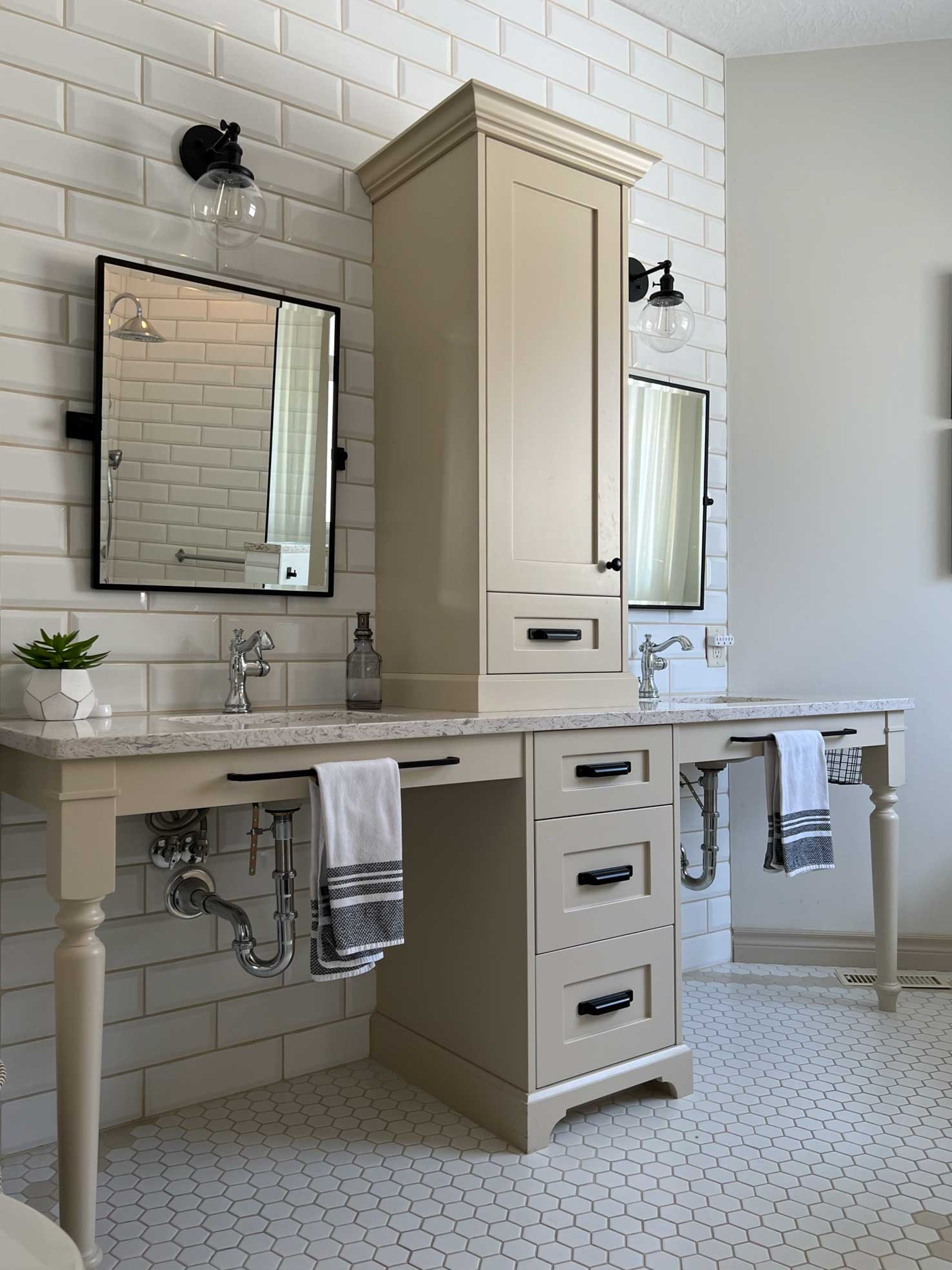This photograph depicts a meticulously staged his-and-hers bathroom in portrait orientation. The bathroom features two sinks set into a luxurious granite or possibly tannish marble countertop, separated by a tall tan cabinet that stretches upward. Each sink is paired with its own black-framed rectangular mirror and a light fixture mounted above. The sinks are equipped with shiny silver metallic faucets and are accompanied by decorative items such as a soap dispenser and a small plant in a white bowl. 

In front of each sink hangs a bath towel over a black bar. Below the countertop, the space reveals the exposed plumbing and is supported by a beige painted wooden base with drawers that feature black handles. The walls are adorned with white subway tiles, and the floor is covered in tiny hexagonal ceramic tiles, some of which form a tan stripe, adding to the bathroom's clean and elegant aesthetic. The overall design showcases a blend of modern and functional elements, making it suitable for both a hotel and a high-end residential setting.